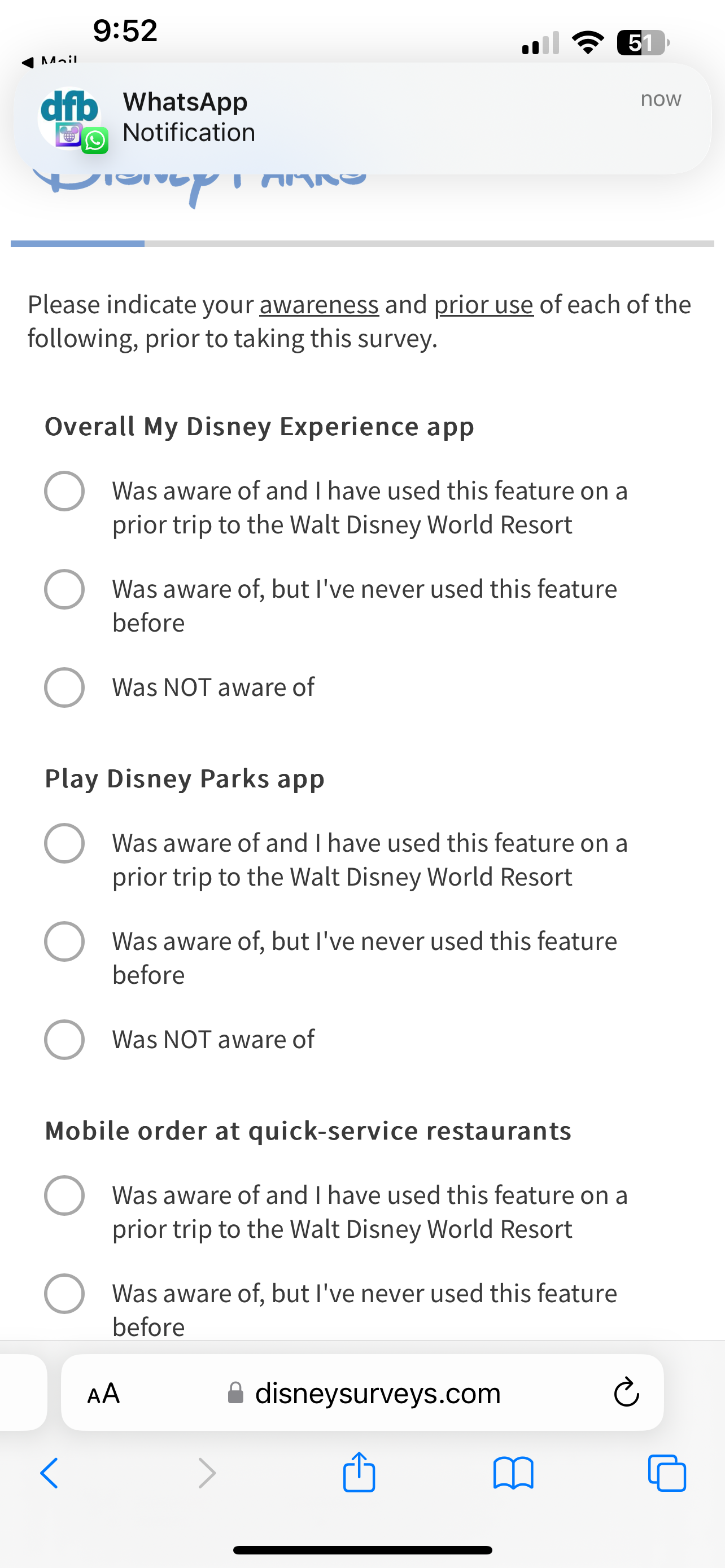A screenshot from a mobile device displays a comprehensive survey from the My Disney Experience app concerning user familiarity and previous usage of various features at the Walt Disney World Resort. The survey asks participants to indicate their awareness and prior use of the Disney Experience App, Play Disney Parks App, and Mobile Order at quick service restaurants, each with options: "Aware and have used," "Aware but have not used," and "Not aware."

The screen includes elements like a blue refresh button, a blue back arrow, and a gray forward arrow, with additional buttons for upload and navigation. The interface displays traditional survey design elements on a white background, black horizontal lines, and blue tabs.

The notification bar at the top of the screen shows a WhatsApp notification icon with the initials "DFB" inside a green square featuring a rotary phone, a Wi-Fi symbol, a partially filled battery icon at 51%, and the time. Disney-themed graphics, including a Mickey Mouse head, are also visible.